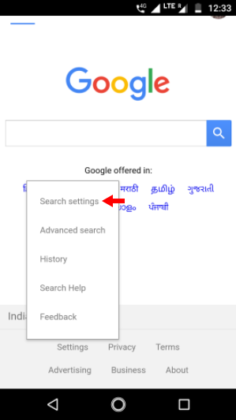The image depicts a smartphone screen with various interface elements. At the top, there is a long black status bar. To the right, there is an icon of a white phone, followed by the text "4G," and immediately after, a triangle pointing left beside the label "LTE." Adjacent to these, a battery icon shows a low charge with its lower half in white. The time displayed is 12:33.

Below the status bar, the word "Google" is prominently displayed in its usual colors: G-O-O-G-L-E. Next to this is a long search bar, alongside a blue square containing a white magnifying glass icon.

Further down, the text "Google offered in" is visible, followed by a clickable link labeled "Search settings" accompanied by a right-pointing arrow meant to highlight this option. Additional clickable options listed are "Advanced search," "History," "Search help," and "Feedback."

Towards the bottom of the screen, horizontally-arranged text links read "Settings," "Privacy," and "Terms." Below this line, there are more options, including "Advertising," "Business," and "About." Finally, at the very bottom, a long black line is present, containing a left-pointing arrow, a white circle, and to the right of that, a white square.